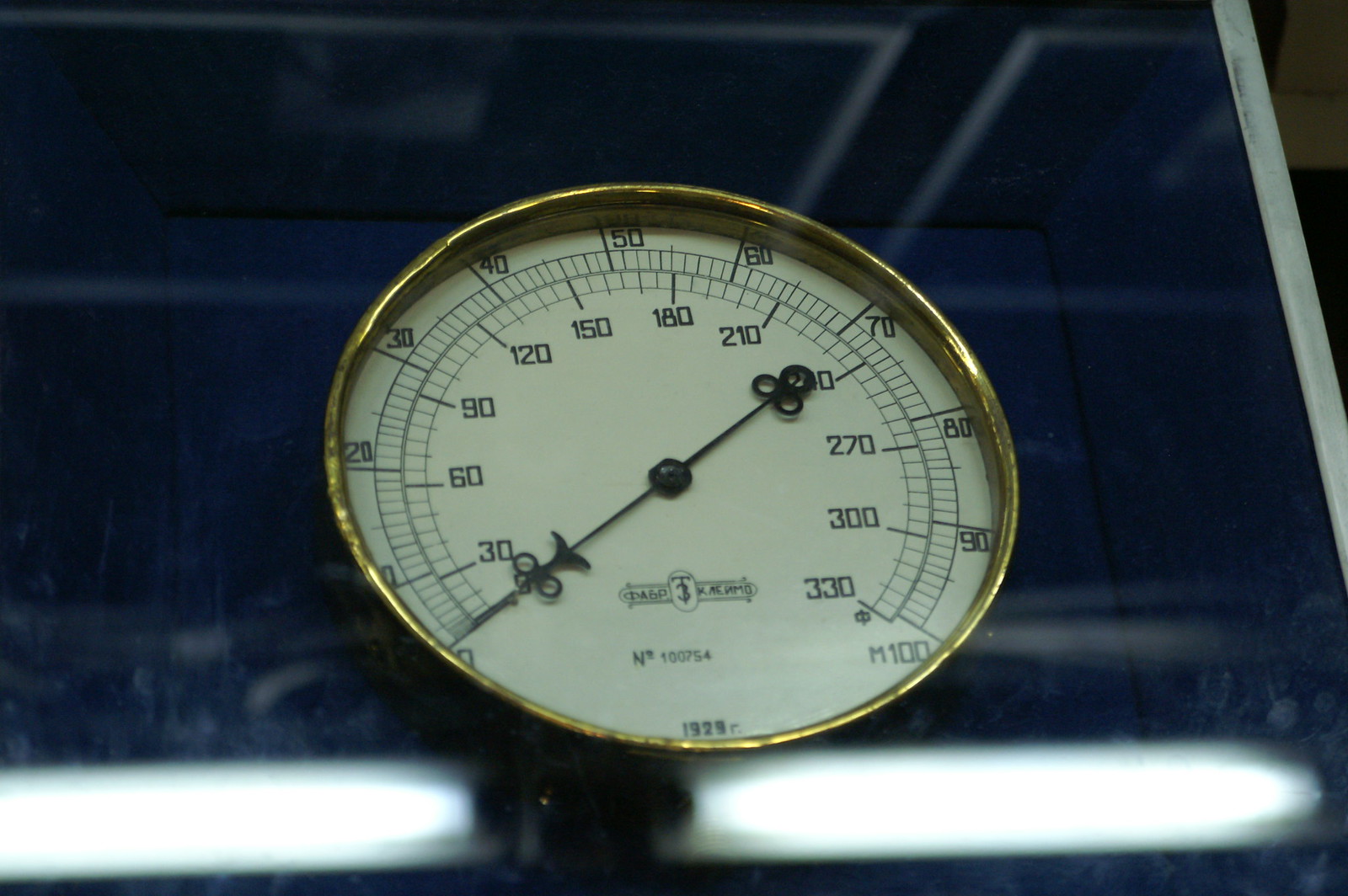This photograph features a sophisticated gold speedometer, prominently centered. The speedometer itself is distinguished by its golden rim and a pristine white base, adorned with black markings and a sleek black dial. The instrument displays an inner circle scale ranging from 0 to 330, while the outer circle ranges from 0 to 100. Encasing this precision device is a dark blue housing, which appears to be constructed from metal or steel, reflecting its robustness. The glass cover of the case exhibits reflections of fluorescent ceiling lights, indicating that the image was captured in a well-lit indoor setting. The speedometer is meticulously centered, although the entirety of the blue case is not fully visible, with some edges slightly cut off in the frame.